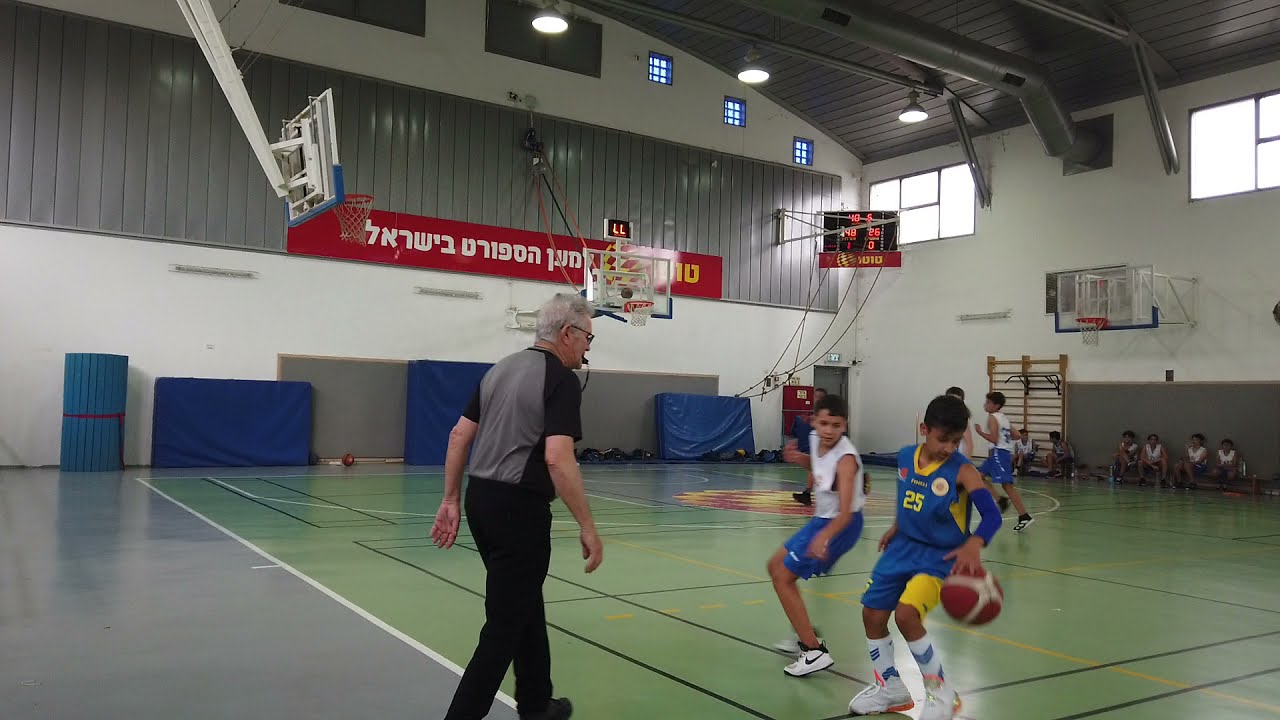This vibrant, full-color photograph captures an engaging youth basketball game inside a gymnasium during the daytime, as suggested by the brightly lit windows. The gym features white walls and a gray, arched ceiling with visible piping, and the floor transitions from gray cement on the left to a green basketball court on the right. Multiple basketball hoops extend from the walls, creating a well-equipped sports arena. In the foreground, an older Caucasian referee with gray hair, black glasses, and a whistle stands attentively, clad in a black and gray short-sleeved shirt and black pants. He observes two young boys with light brown skin: one dribbling with his left hand while wearing a blue and yellow sleeveless uniform numbered 25, and another guarding him in a white sleeveless jersey and blue shorts. In the background, additional players are practicing, and a line of students is seated on a bench along the far right-hand wall. There is a sense of international ambiance owing to a red banner with white, non-English script adorning the back wall. The scoreboard reveals a score of 48 to 26, highlighting the competitive nature of the game.